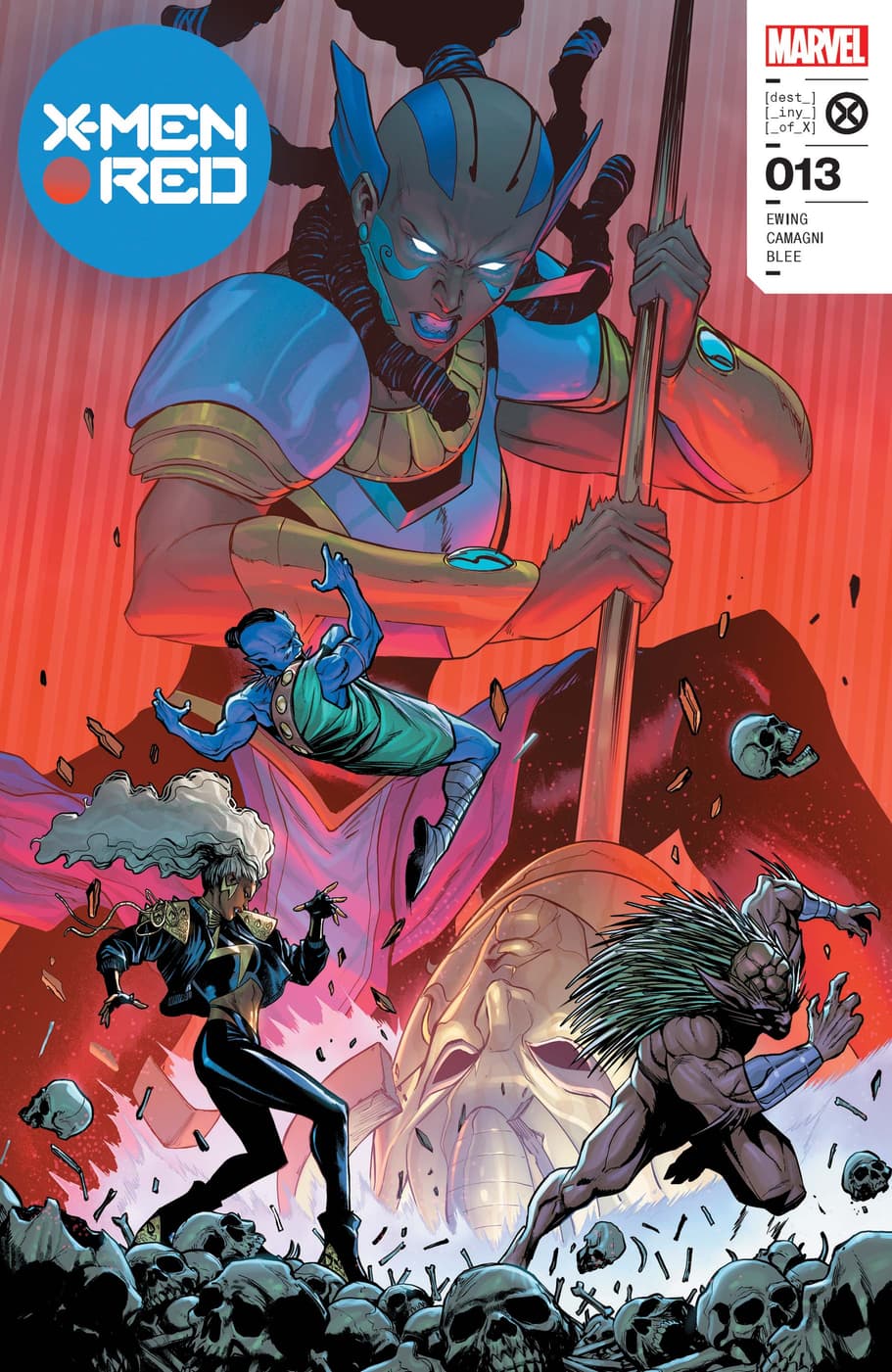The cover of the comic book, titled "X-Men Red," has vibrant and dramatic artwork. In the upper left corner, a blue circle with white text reads "X-Men Red," accentuated by a smaller red circle. On the upper right, the characteristic Marvel logo is prominent, featuring white letters against a red rectangle background. Below it, the title "Destiny of X" is mentioned, with a black X inside a circle.

Dominating the scene is a fierce, menacing woman with dark skin adorned in blue and gold armor. Her hair is thick, chunky dreadlocks wrapped with blue bands, and her head is gray with striking blue stripes and blue fins extending from the sides. Her glowing blue eyes add intensity to her intimidating presence. She wields a staff-like weapon that has a face on its yellow, shovel-like head, which she thrusts into the ground covered in a pile of skulls.

Flanking her are two distinct creatures: one, a beast-like entity with brown, spiky hair and dark skin, and the other, a female figure in a black, tight outfit with long white hair, likely the X-Men character Storm. In the center, a blue, demon-like figure appears to be falling amidst a backdrop that bursts with vibrant orange and red hues, enhancing the chaotic and dramatic atmosphere of the scene.